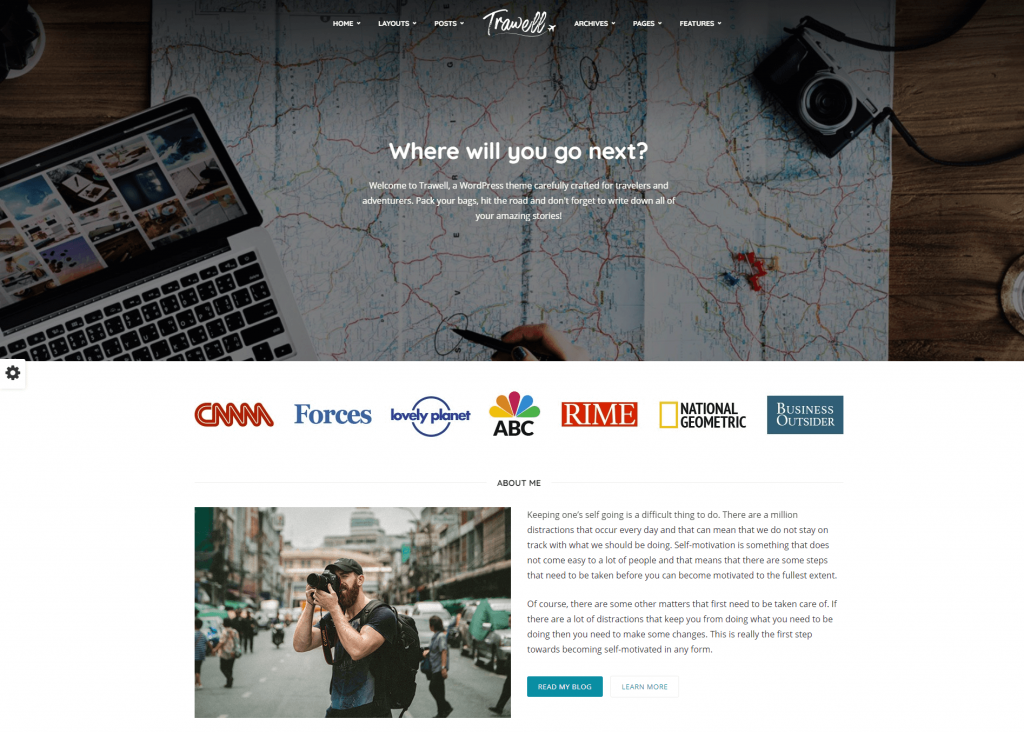A sleek, business-like travel webpage titled "Travell" is prominently displayed on a laptop surrounded by a large map and a camera. The webpage headline poses the question, "Where will you go next?" The laptop screen showcases numerous vibrant images of various travel destinations. Below the pictures, the site features a list of reputable sources such as CNN, Forbes, The Lovely Planet, ABC, RIME, National Geographic, and Business Outsider, suggesting high credibility and wide recognition. Additionally, there is an "About Me" section with a photo of a gentleman holding a camera, surrounded by a busy urban scene. The text under this section is in small font, making it difficult to read. Overall, the webpage exudes a professional yet inviting atmosphere, likely appealing to a broad audience of travel enthusiasts.